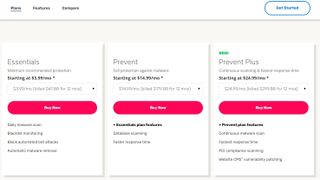The screenshot presents a visually structured interface with a white bar spanning the top, featuring three tabs that are too small to read. At the top-right corner of the bar, there is a blue circular button with some text inside it. Below the white bar, the background transitions to a cream color and displays three equally sized rectangular sections, which are slightly taller than they are wide.

Centered within each of these rectangles is a prominent red button that spans almost the entire width of the rectangle, bearing white text. Each section has a title positioned at the top, reading "Essentials," "Prevent," and "Prevent Plus" from left to right. Above the "Prevent Plus" section, there is a "NEW" label in bright green letters. Each section also contains some smaller text above their respective red buttons, followed by three lines of very small, minimized print at the bottom, which is difficult to read. The entire interface appears wider than it is tall, suggesting that it might continue beyond what is visible in the screenshot, particularly if viewed on a larger screen such as a computer monitor.